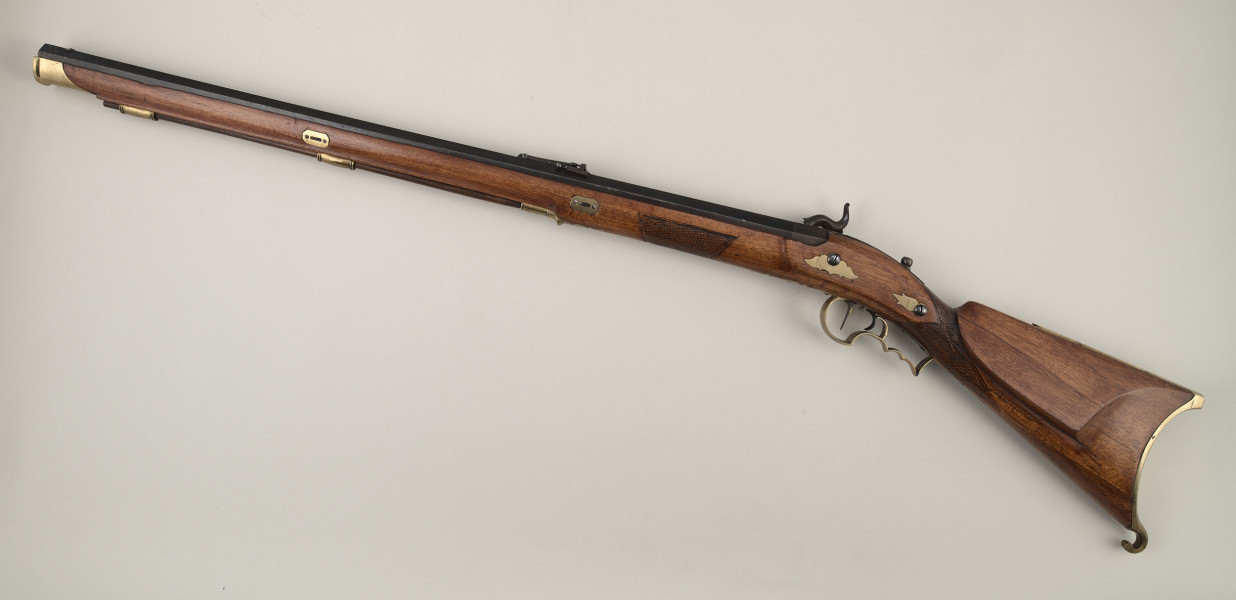The image showcases an antique rifle, possibly a musket, that exudes an aura of historical craftsmanship. The lengthy firearm, approximately three to four feet, is predominantly constructed from darker-hued wood, indicating its vintage nature, likely over a century old. Adorning the rifle are intricate gold or bronze-colored metal furnishings, including a notable gold trigger and several gold pieces underneath. The upper part of the rifle is distinct with a continuous black metal strip running from the butt to the muzzle. The butt of the rifle features a silver end piece with a small hook, and a prominent gold fixture adds to its ornate design. Towards the back of the rifle, delicate engravings decorate the wood, enhancing its classic look. The firearm is positioned on a solid white table surface, against a contrasting gray wall, emphasizing its refined and well-preserved condition.